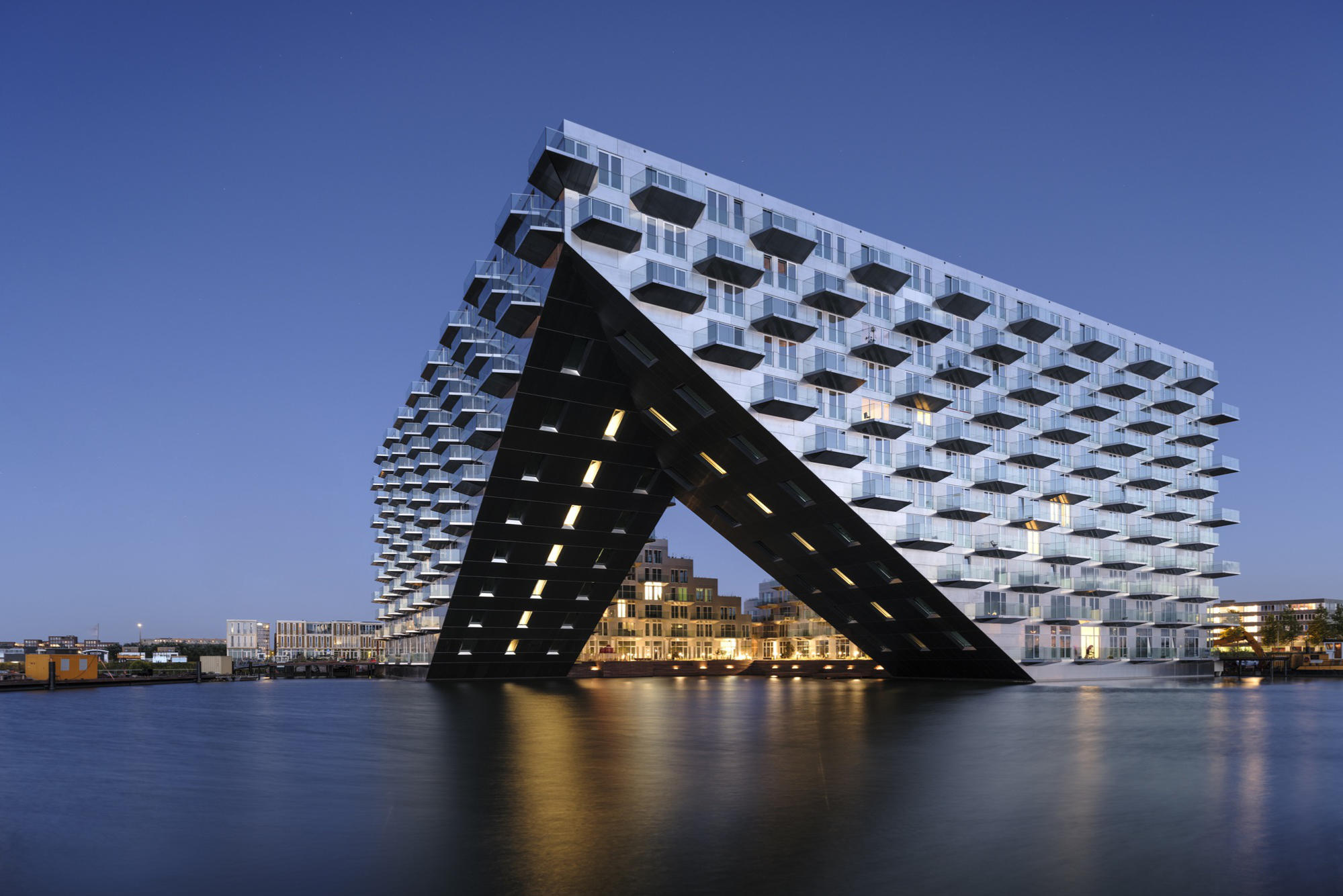This color photograph features an elaborate, futuristic-style building, likely an architectural rendering of a high-end apartment complex or hotel, situated on a tranquil body of water. The sky is a deep, dark blue, indicative of dusk. The striking structure juts out over the water, forming an inverted V or arrow shape with a distinct, triangular cutout at its center. This cut-out area, illuminated by lights, reveals other parts of the building and possibly a dock below. The building’s facade gleams with shiny steel and reflective glass, creating a mirrored effect that enhances its modern aesthetics.

The building ascends to 11 stories, with more rooms on the upper floors than the lower floors due to an overhang design. Each room appears to have a balcony, though it's ambiguous whether these are open or enclosed. The calm, blue water below enhances the sense of serenity and luxury of the location, which might be a resort area. Surrounding the main structure are other industrial or modern warehouses, further emphasizing the advanced, architectural feel of the scene. No people, animals, or writing are visible in the photograph, keeping the focus entirely on the impressive building and its surroundings.